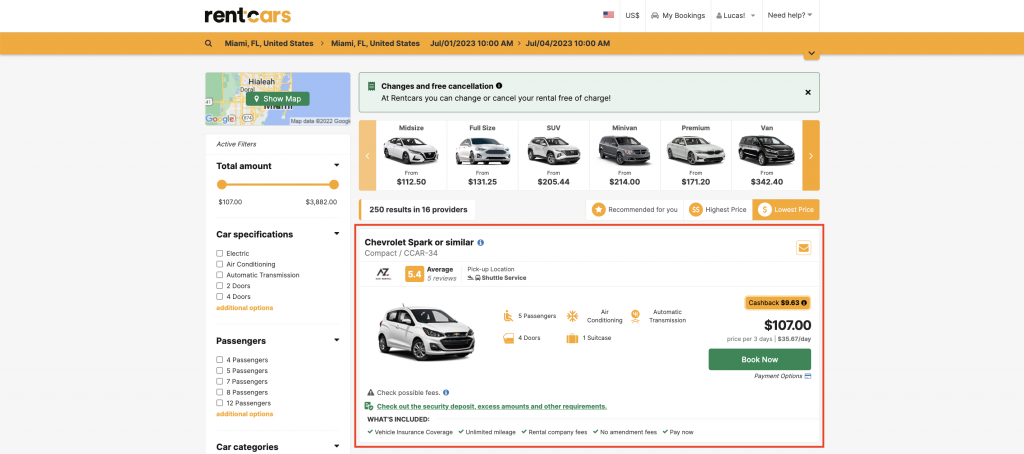**Detailed Caption for Car Rental Website Screenshot:**

This screenshot captures the homepage of a car rental website. At the top, the site's header is prominently displayed with a black and gold theme, featuring the title "Rent Cars." Adjacent to the title are an American flag icon, the word "US" accompanied by a dollar sign, tabs labeled "My Bookings," "Lucas," and a "Need Help" option.

Just below the header, there is a noticeable orange search bar specifying "Miami, Florida, United States" as the pickup and drop-off location. The rental period is indicated as from July 1, 2023, at 10 a.m. to July 4, 2023, at 10 a.m. To its left, a small rectangular inset displays a map of the specified location.

Beneath this section, there are several filter options to refine the car search based on preferences and specifications. These filters include categories like "Electric," "Air Conditioning," "Automatic Transmission," "Two Door," "Four Doors," and other additional options. For passenger capacity, choices range from "Four Passengers" up to "Twelve Passengers."

Further down, under the "Car Categories" section, a selection of six different car options is showcased, each listed with their price options. On the right side of the screen, a specific car option is highlighted within a red box. This option is the "Chevrolet Spark or similar," accompanied by an image of a white car with a black interior. Next to the car image, several pieces of important information are provided: a cashback offer of $963, a highlighted price of $107 in a yellow bar, and a green "Book Now" button to proceed with the rental booking.